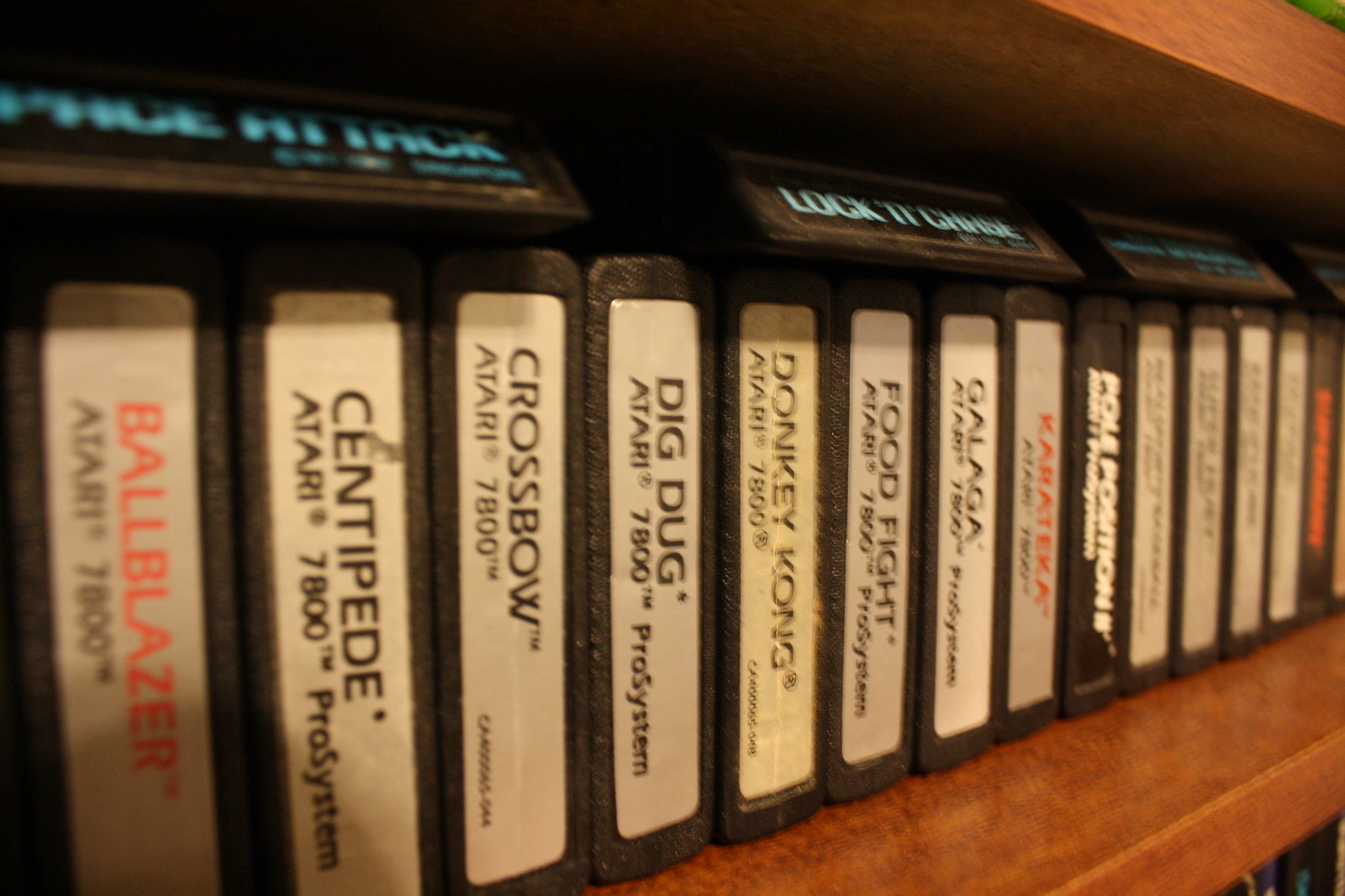This photograph showcases a large, meticulously arranged collection of old Atari 7800 game cartridges on a highly polished, medium-grain wooden shelf. Each game is displayed with the recognizable Atari logo and most have white labels with black lettering, though some titles feature red-orange text or black backgrounds. The clearer titles among the visible games include Ballblazer, Centipede, Crossbow, Dig Dug, Donkey Kong, Food Fight, Galaga, and Karateka, with several in the distance becoming harder to discern due to blurriness. Above the main row of cartridges, which are all black, there are additional blurry signs with blue lettering, possibly indicating more games or game-related information. The shelf also appears to hold multiple rows of video games, suggesting a richly stocked collection that extends beyond what is immediately visible.